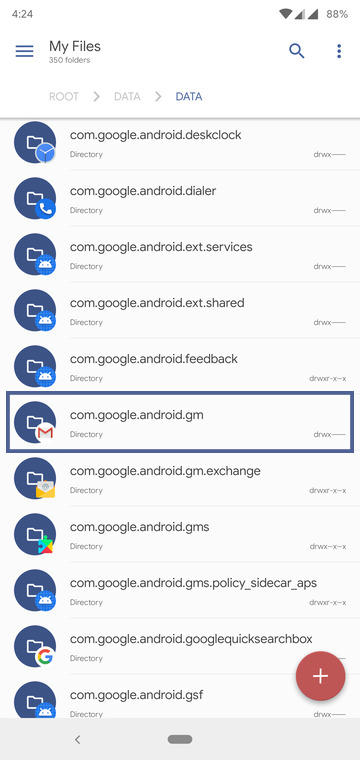In this portrait-mode screenshot, presumably taken from a phone, we observe a file directory interface with a predominantly off-white background. 

Starting from the top left, the status bar displays "424" on the left side and the battery level "88%" on the right. The subsequent row features a menu icon, represented by three blue horizontal lines, followed by the title "My files" and a count indicating "350 files/folders." On the far right, a search icon and a menu denoted by three dots are visible.

The third row starts with a breadcrumb navigation path showing “root > data > data,” with the latter “data” highlighted in blue, while the preceding terms are in gray. Directly below, a horizontal gray stripe spans the width of the screen.

The primary content section displays five distinct rows, each beginning with a large blue circle icon on the left, followed by folder names. The rows list directories such as:

1. `com.google.android.desktop directory` (with a clock icon)
2. `com.google.android.dialer directory` (with a phone icon)
3. `com.google.android.extensionservices directory` (with an Android icon)
4. `com.google.android.extensionshare directory` (with an Android icon)
5. `com.google.android.feedback directory` (with an Android icon)

Highlighted in blue is the `com.google.android.gm` directory, marked by a large blue rectangle encompassing the Gmail icon (a white envelope). Below this, it reads "directory," and on the bottom right corner of the highlighted area, the permissions `drwx` are indicated.

At the bottom right, a rounded button with a plus sign awaits user interaction.

This detailed screenshot reflects a methodical navigation through a phone's file system, exemplifying both structure and organization within the file hierarchy.